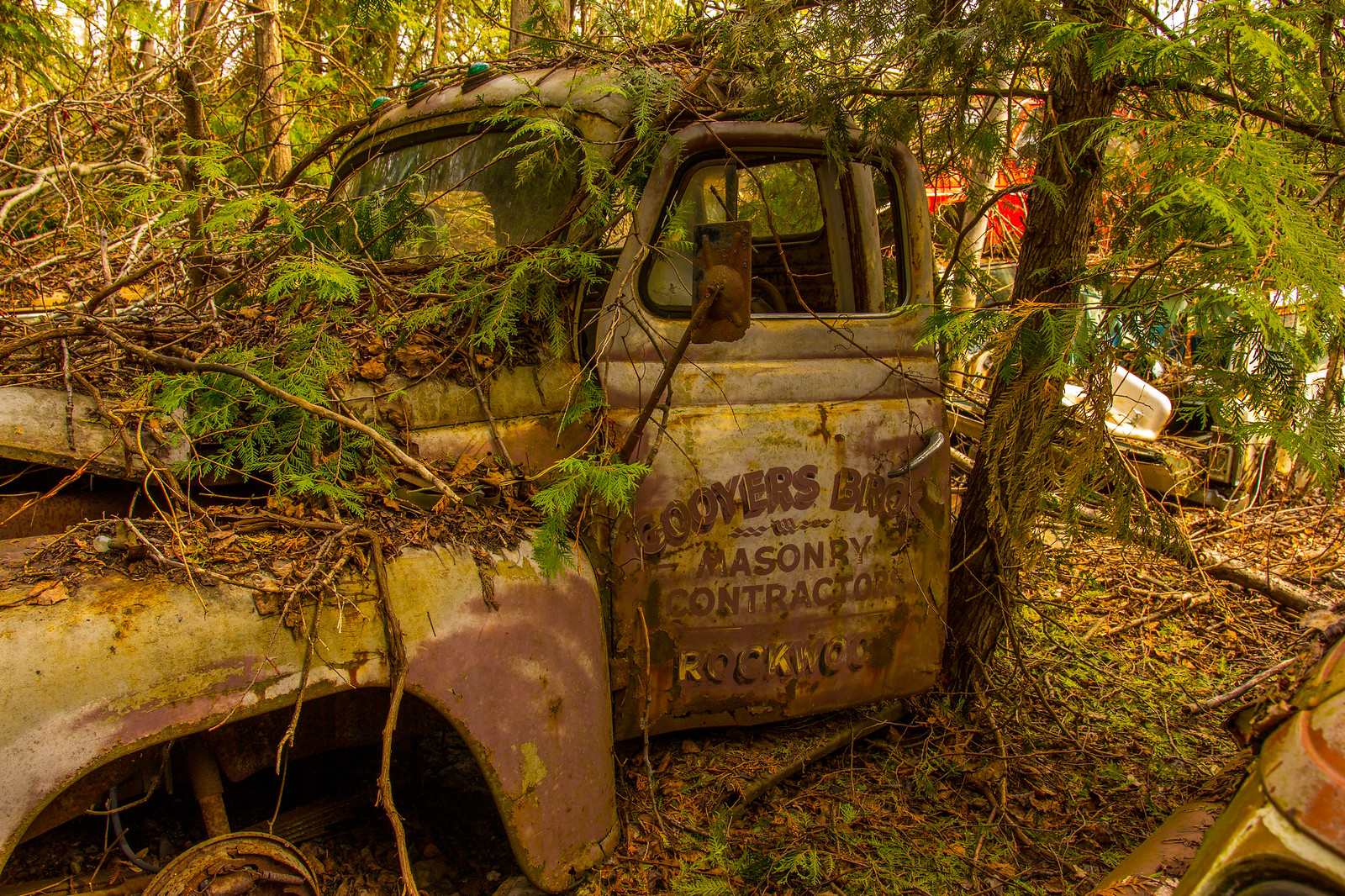This photograph, taken in an outdoor setting, showcases the front end of a decaying, rusted truck cab amidst a dense forest environment. The vehicle, likely a pickup truck, is enveloped by greenery, with vines, plants, and moss growing over and around it. Dried leaves and branches lay scattered on top and across the hood, and green pine needles and brown dirt are visible beneath it. The truck is extensively rusted, giving it a predominant brown color, although remnants of its original white paint persist. The door of the truck is notably open, and a faint side view mirror clings to the cab. A faded advertisement on the door reads, "Coors/Mason by Contractor Rockwood," though it is partially obscured by rust and grime. The front left tire is missing, and the hood is slightly ajar. Surrounding the truck, more trees and assorted pieces of machinery are discernible, enveloped by the untamed forest, emphasizing the truck's long abandonment.